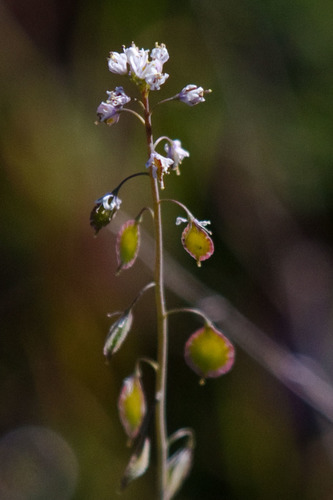The image is an up-close photograph of a plant showcasing a mix of blooming and budding flowers against a blurred background. The background features soft hues of green, white, and hints of pink and yellow, along with the faint outline of a stick or branch. Dominating the forefront is a slender plant stem, about the thickness of a pencil, extending from the bottom to almost the top of the picture. Along the stem, staggered on either side, are drooping leaves with a central yellow coloration surrounded by pink edges, each tipped with a small notch. Progressing upwards, you encounter tiny, bell-shaped white buds. Higher up on the stem, the flowers appear partially bloomed with delicate white petals tinged with purplish hues. There are approximately five or six small petals at the top and further down the stem, with leaves interspersed in between. Overall, the image captures a detailed progression of the plant's growth stages with a soft, blurred mix of greens and browns in the background, emphasizing the intricate details of the stem and budding leaves.